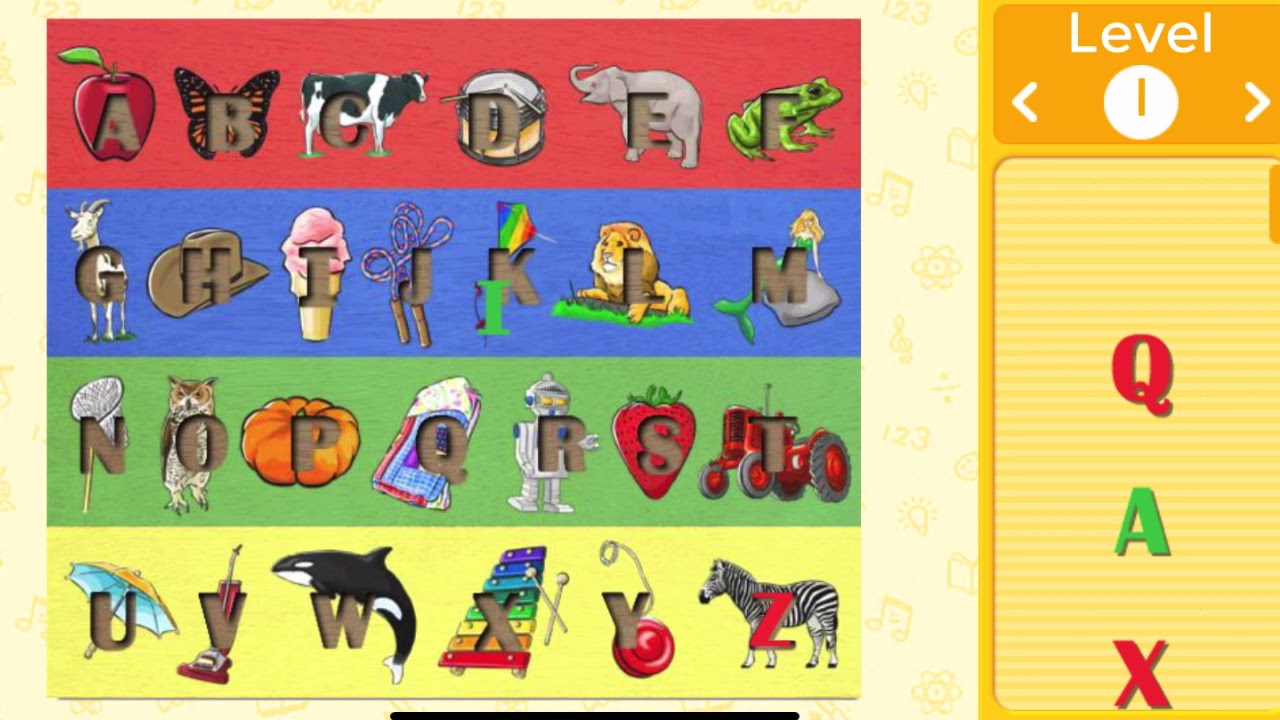The image depicts a colorful and engaging website designed to resemble a children's toy that teaches the alphabet. Each letter from A to Z is represented by an empty slot where wooden blocks can be placed. Behind each slot is an illustration of an object that corresponds to the respective letter. Specifically, A is for Apple, B is for Butterfly, C is for Cow, D is for Drums, E is for Elephant, F is for Frog, G is for Goat, H is for Hat, I is for Ice Cream, J is for Jump Rope, K is for Kite, L is for Lion, M is for Mermaid, N is for Net, O is for Owl, P is for Pumpkin, Q is for Quilt, R is for Robot, S is for Strawberry, T is for Tractor, U is for Umbrella, V is for Vacuum Cleaner, W is for Whale, X is for Xylophone, Y is for Yo-Yo, and Z is for Zebra. The website is divided into four color-coded sections: letters A through F have a red background, G through M have a blue background, N through T have a green background, and U through Z have a yellow background, making it easy for kids to identify different segments of the alphabet.